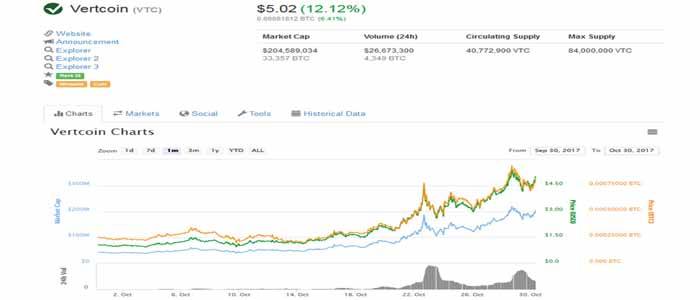This is an image showing a detailed screenshot of Vertcoin's financial data, specifically illustrating its market performance. The screenshot is landscape-oriented and lacks defined borders, set against a faint grey rectangular background.

In the upper-left corner, there is a green circle with a white checkmark inside, next to black text reading "Vertcoin," followed by the ticker symbol "VTC" in grey parentheses. Centered at the top, the current price is prominently displayed as $5.02 in black, with a green percentage figure of 12.12%, indicating a likely increase.

Below "Vertcoin," there are various clickable links highlighted in blue, including "Website," "Annual Statement," and "Explorer," among others that are less legible. Underneath the price, columns categorize essential financial metrics: "Market Cap," "Volume," "Circulating Supply," and "Max Supply," each accompanied by relevant data.

The central part of the screenshot presents a detailed graph, featuring intersecting blue, green, and yellow lines representing different market trends. The axes are marked in green and black, with some orange highlights on the side. The title "Vertcoin Charts" is visible, along with sorting options such as by day, month, years, year-to-date, and total performance.

At the top of the interface, there are navigation options for viewing "Charts," "Markets," "Social," "Tools," and "Historical Data," with "Charts" currently selected and enclosed in a grey border. The comprehensive layout and vibrant colors provide an in-depth look into Vertcoin's market dynamics.